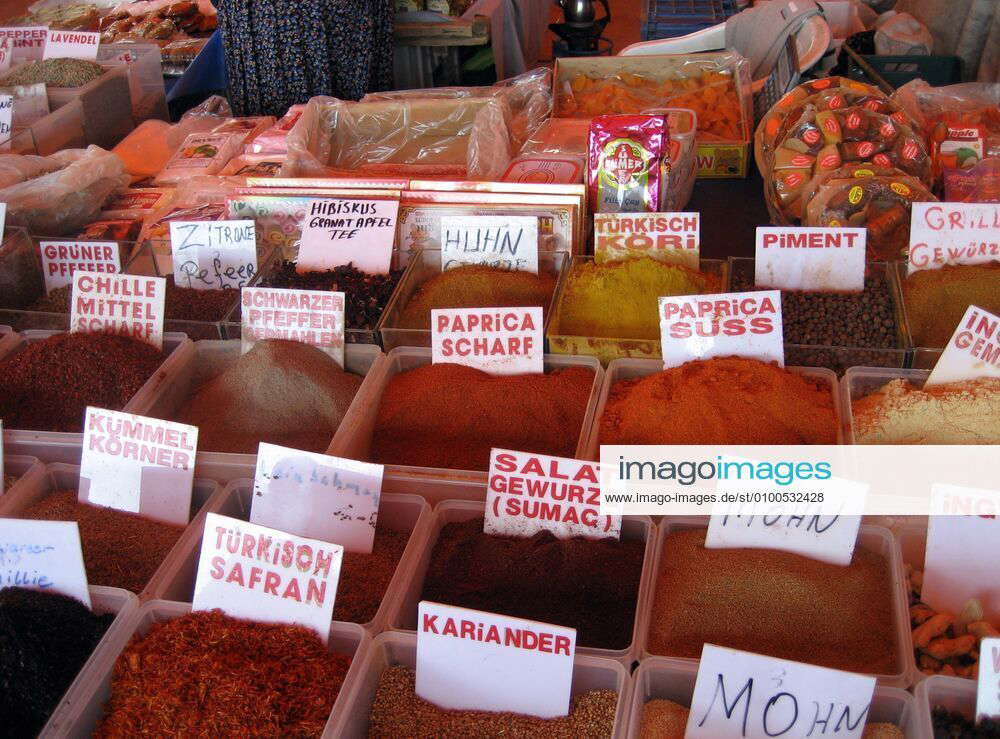This image captures a vibrant and bustling Middle Eastern or Asian spice market, showcasing a rich variety of herbs and spices laid out across a table. The table is filled with rows of loose spices organized in wooden boxes, each marked with a white sign indicating the type. From front to back, visible spices include Turkish saffron, coriander, kamelkorner, sumac, chili, schwarzer pepper, scharf paprika, paprika sauce, grunner puffer, citrine, hibiscus tea, Turkish coriander, piment, and grill. The spices exhibit a spectrum of colors, from deep reds and bright yellows to earthy greens and subtle browns. Along the right, the spices are arranged in a grid, five boxes across and four deep, with each section carefully labeled. Above these spices, the upper part of the image shows additional market goods, including plastic packaging and various items like a lantern and a chair, suggesting an eclectic market setting. The marketplace appears to be outdoors or in a semi-open area, likely a roadside or shopping district, with a combination of rustic charm and chaotic liveliness indicative of a traditional spice bazaar.